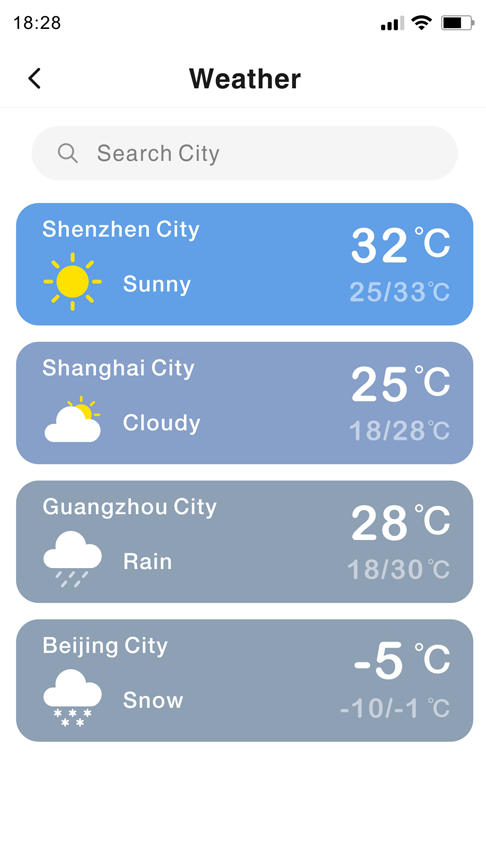The image showcases a smartphone displaying a weather application. The phone's battery is approximately three-quarters full, and the connection strength is strong, indicated by three out of four bars. The time, set in military format, reads 18:28. At the top of the screen, in bold black lettering, the word "Weather" is prominently displayed with a left-facing arrow beside it. Below "Weather," there is a light gray bar spanning the width of the screen.

Just beneath this bar is a search field, also light gray, with placeholder text that reads "Search city" accompanied by a magnifying glass icon. The first city displayed in the weather information is Shenzhen, highlighted in blue with a current temperature of 32°C. The forecast shows a high of 25°C and a low of 33°C, with clear, sunny conditions illustrated by a full sun icon.

Following Shenzhen is Shanghai, listed in a lighter blue color indicating partly cloudy weather, represented by a sun and cloud icon. The temperature is 25°C, with a range from a high of 18°C to a low of 28°C. Next is Gansu City, shown in gray, featuring rainy weather with a cloud and raindrops icon. The current temperature is 28°C, with a high of 18°C and a low of 30°C.

At the bottom of the list is Beijing, which has snow conditions depicted by a cloud with snowflakes. The temperatures range from a current -5°C to a high of -10°C and a low of -1°C.